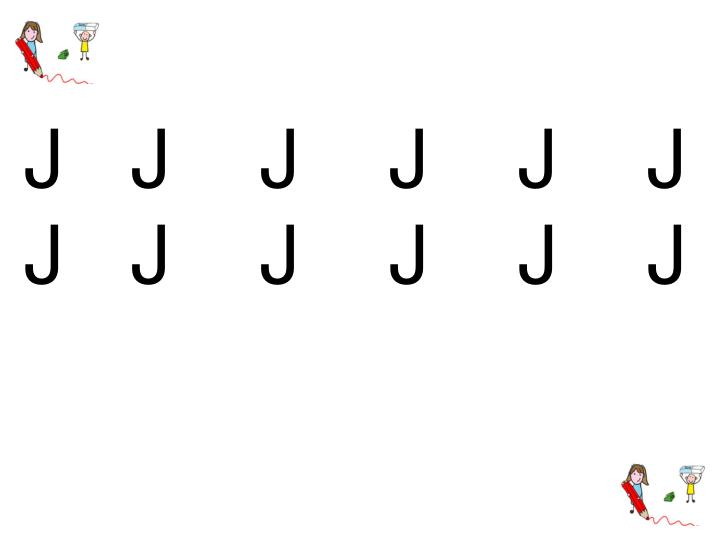This image appears to be an instructional illustration likely designed for a child's educational book. The main background is white, featuring the capital letter 'J' repeated 12 times in a sans serif font, arranged in two rows of six. In both the upper left-hand corner and the lower right-hand corner, there is a charming hand-drawn cartoon of a little girl and a boy. 

The girl, with brown hair and clad in a blue shirt, is holding an oversized red pencil, as tall as she is, drawing a squiggly red line on the ground. Beside her stands a blonde boy in a yellow shirt, lifting a large blue and white eraser above his head. Notably, a small green object is positioned between them on the ground. The illustration in the upper left-hand corner is mirrored exactly in the lower right-hand corner, adding a whimsical repetitive element to the image.